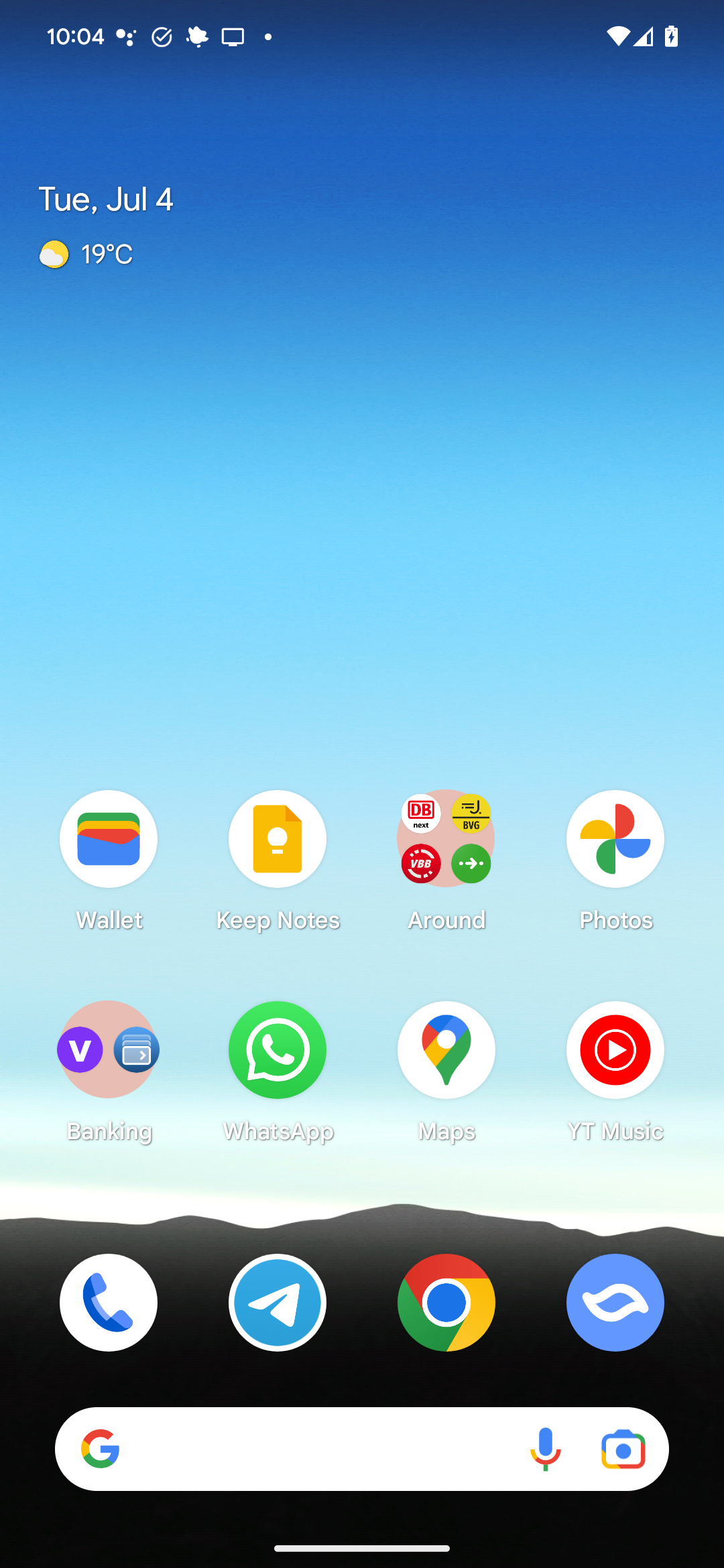A screenshot of a home screen on an Android cell phone. At the top of the screen, the status bar displays the current time alongside various icons, including those for Wi-Fi connectivity and battery level. The background image features a scenic mountain range, with rugged peaks at the bottom transitioning to a sky that extends to the top of the screen. The date is noted as Tuesday, July 4th, and the weather information indicates partly cloudy conditions with a temperature of 19 degrees Celsius.

The main portion of the screen is populated with several app icons. These include applications for Wallet, Keep Notes, Photos, Banking, WhatsApp, Maps, and YouTube Music. At the very bottom, there is a multifaceted Google search bar equipped with options to initiate a voice search or use the camera for visual search queries. Additionally, the dock contains essential apps for Phone calls, Messaging, Google Chrome, and another unidentified application.